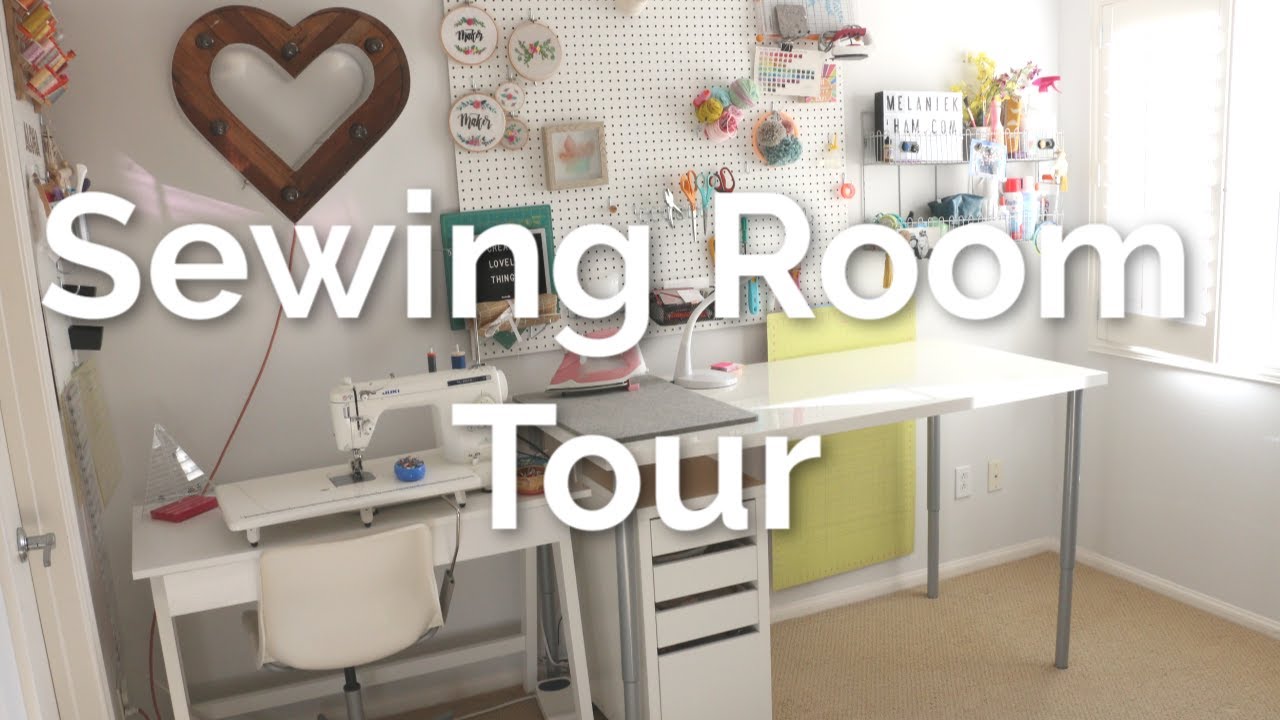The photograph illustrates a well-organized sewing room bathed in ample natural light from a window on the right. Central to the image is a white sewing station featuring a sewing machine and a matching white chair neatly pushed in. Adjacent to this setup, on the right, sits an additional white table supported by two metallic legs, with a white book drawer cabinet underneath and topped by a pink iron and a small gray ironing board. Dominating the back wall, a bulletin board pierced with numerous holes displays an array of sewn items, including circles and squares with images and words, alongside various crafting supplies such as embroidery hoops, pins, needles, yarn, and scissors. Above the sewing machine, a rustic brown heart adorns the wall. Highlighting the scene, bold white text overlay reads "Sewing Room Tour," suggesting this image is part of a guided video exploring different sewing rooms.